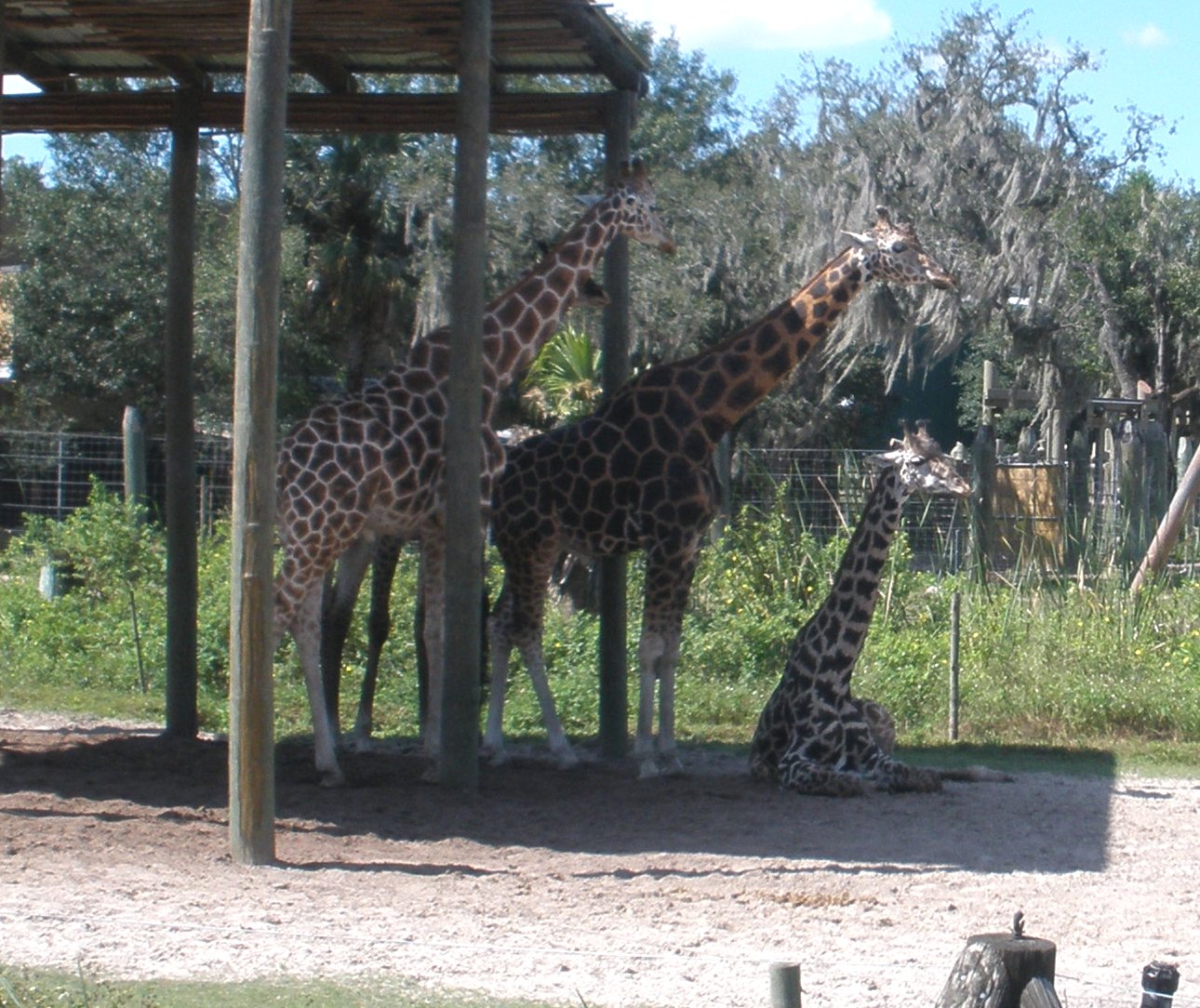This image captures three giraffes in an outdoor enclosure, surrounded by vegetation and a mixture of greenery and dirt. Two adult giraffes are standing while a smaller one sits on the ground. One of the standing giraffes is partly sheltered under a wooden canopy with a roof but no sides, and the other giraffe faces away, positioned halfway under the canopy. The ground is a mix of brown and beige dirt, extending to a lush middle area filled with grass and shrubs. Beyond this, a metal gate separates the enclosure from the larger natural environment, featuring tall trees. The giraffes exhibit varying patterns: the central one with brown spots on a yellowish background, while the others have brown spots bordered by white. The image presents a contrast between the managed enclosure and the wild vegetation beyond.